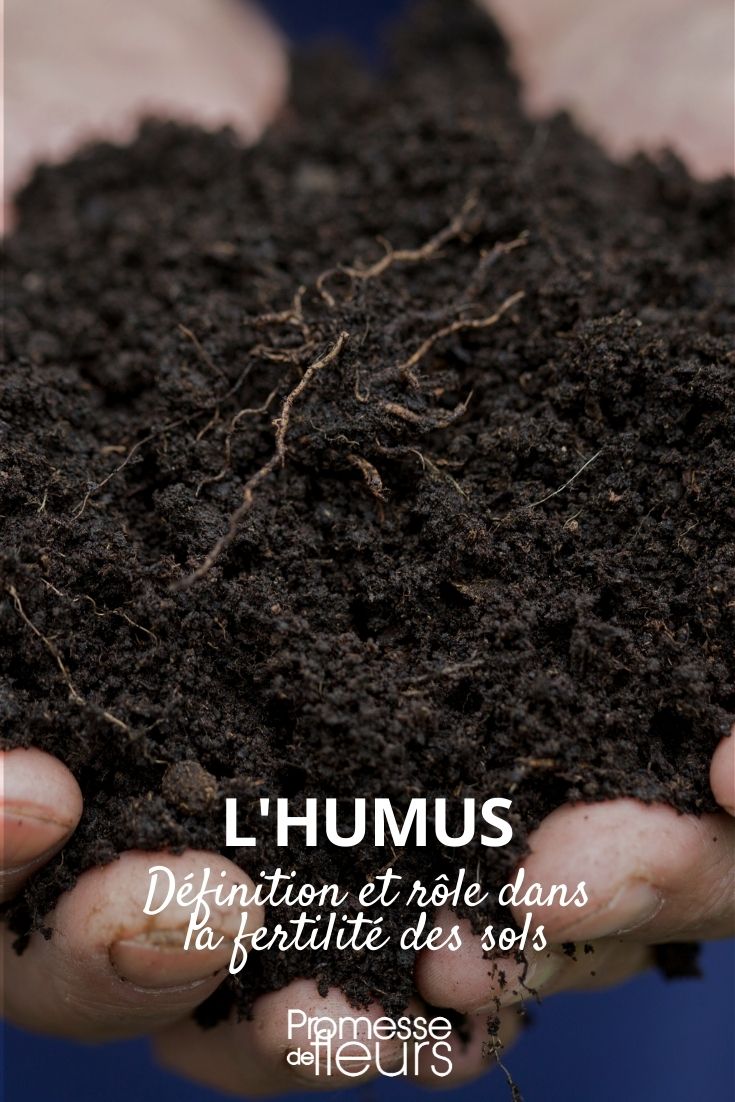The image captures a close-up of two dirty hands holding a moist, dark brown pile of soil, rich with organic matter and roots. The person's fingers are prominently visible at the bottom, slightly soiled with dirt under the nails, gripping the earth firmly. The arms, though slightly blurred and barely discernible in the background, extend underneath the clump of soil, adding depth to the image. White text in French overlays the bottom part of the image, reading "Le Humus: définition et rôle dans la fertilité des sols, promesse de fleurs," which translates to "Humus: definition and role in soil fertility, promise of flowers." The background of the photo has a blue hue, complementing the earthy tones of the soil, and giving the entire scene a poster-like quality.